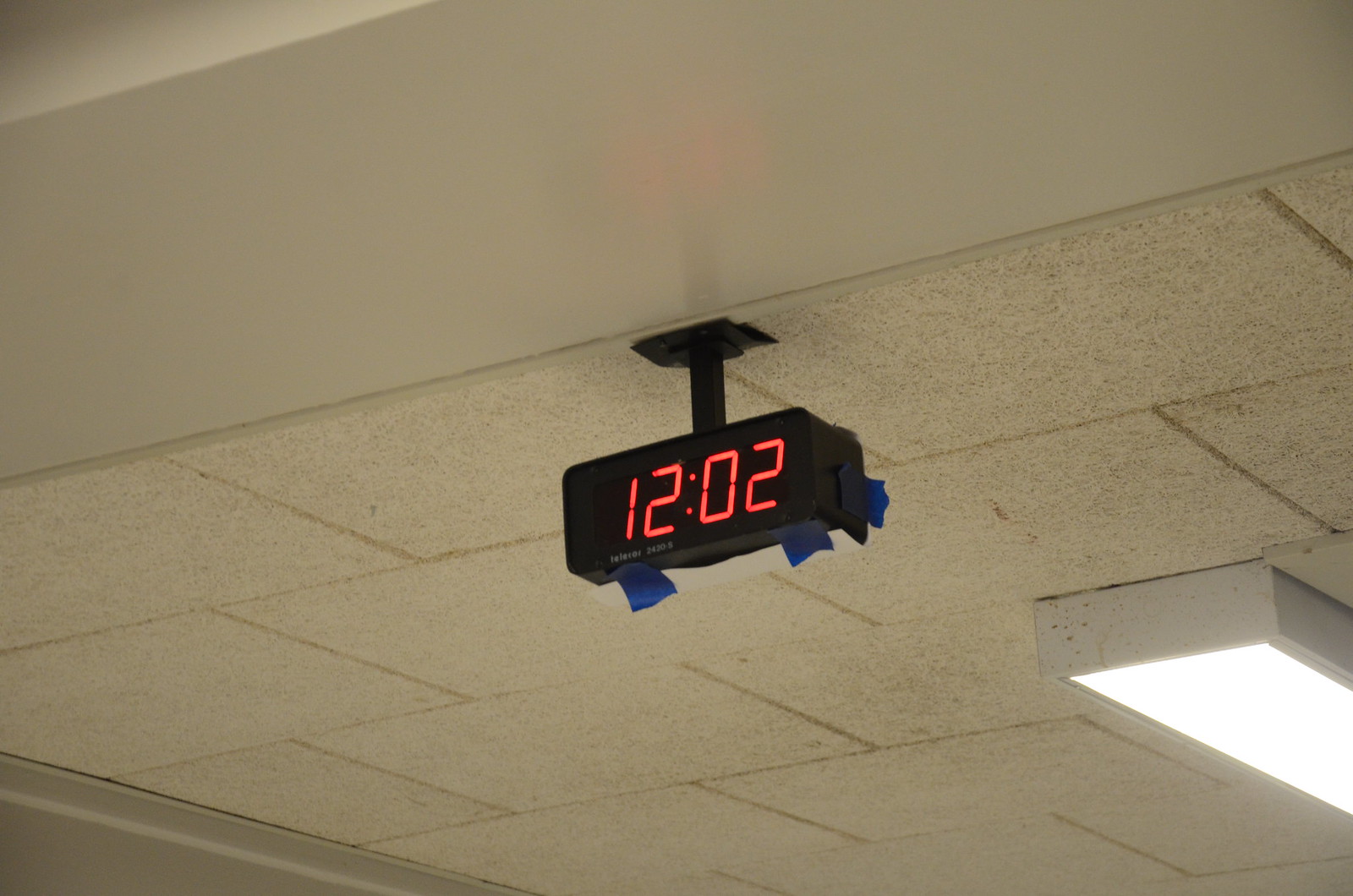This image showcases a digital clock suspended from the ceiling, securely attached amidst visible ceiling tiles. The clock is black with vibrant red numbers, displaying the time as 12:02. It is adorned with three pieces of dark blue tape. Positioned on the edge of a grid of ceiling tiles, the clock is adjacent to a fluorescent light fixture on its right. Notably, the area in front of the clock features a smooth, tile-less expanse of the ceiling, creating a contrasting backdrop.